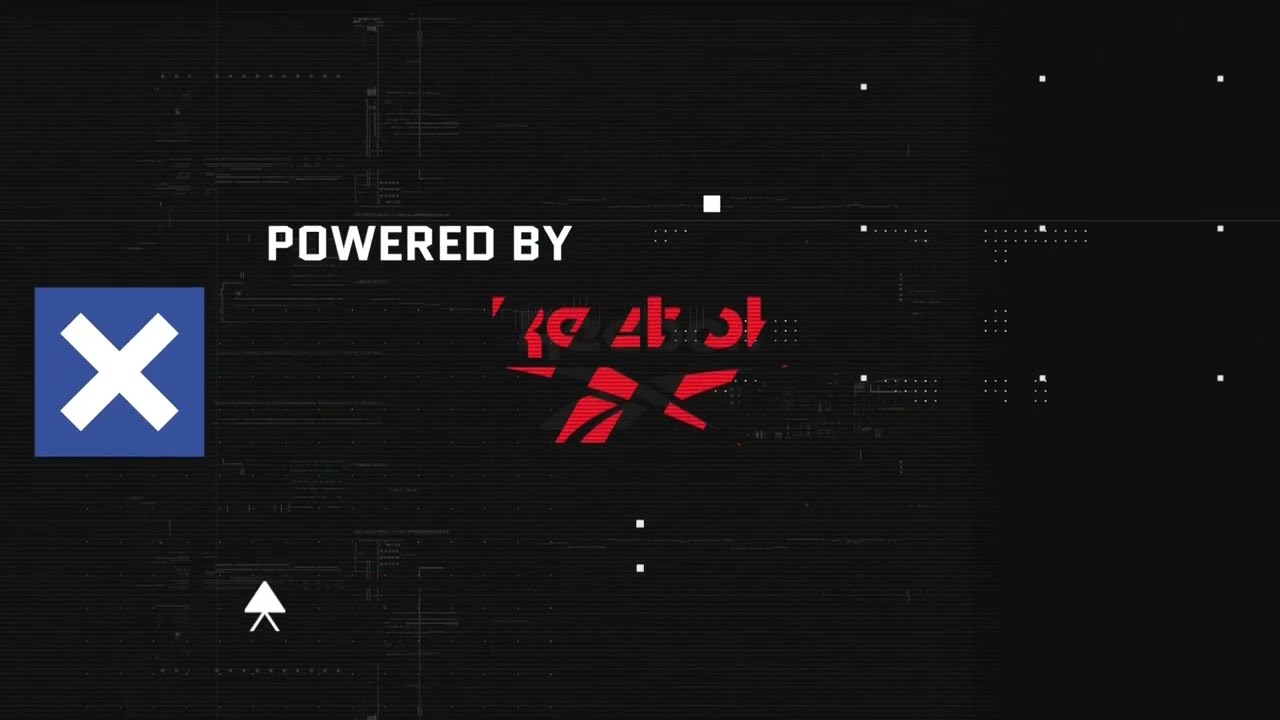The image features a predominantly black background, scattered with tiny white dots, lines, and faint, dark green angles. In the upper right corner, there is a 3x3 grid of evenly spaced white dots. Centered in the lower portion of the image, the word "Reebok" is displayed in red, but it is obscured by three black bars crossing out the lettering. Directly below "Reebok," and slightly to the upper left, is the phrase "powered by" in white letters. Beneath the Reebok logo are two small white dots vertically aligned. On the far left center of the image, there's a blue square with a white X inside it. Near the bottom center, a white arrow points upwards, with small lines extending from its base to the left and right. The overall dark background blends subtly with the additional faded angles, dots, and lines, giving the image a layered, complex graphical design.